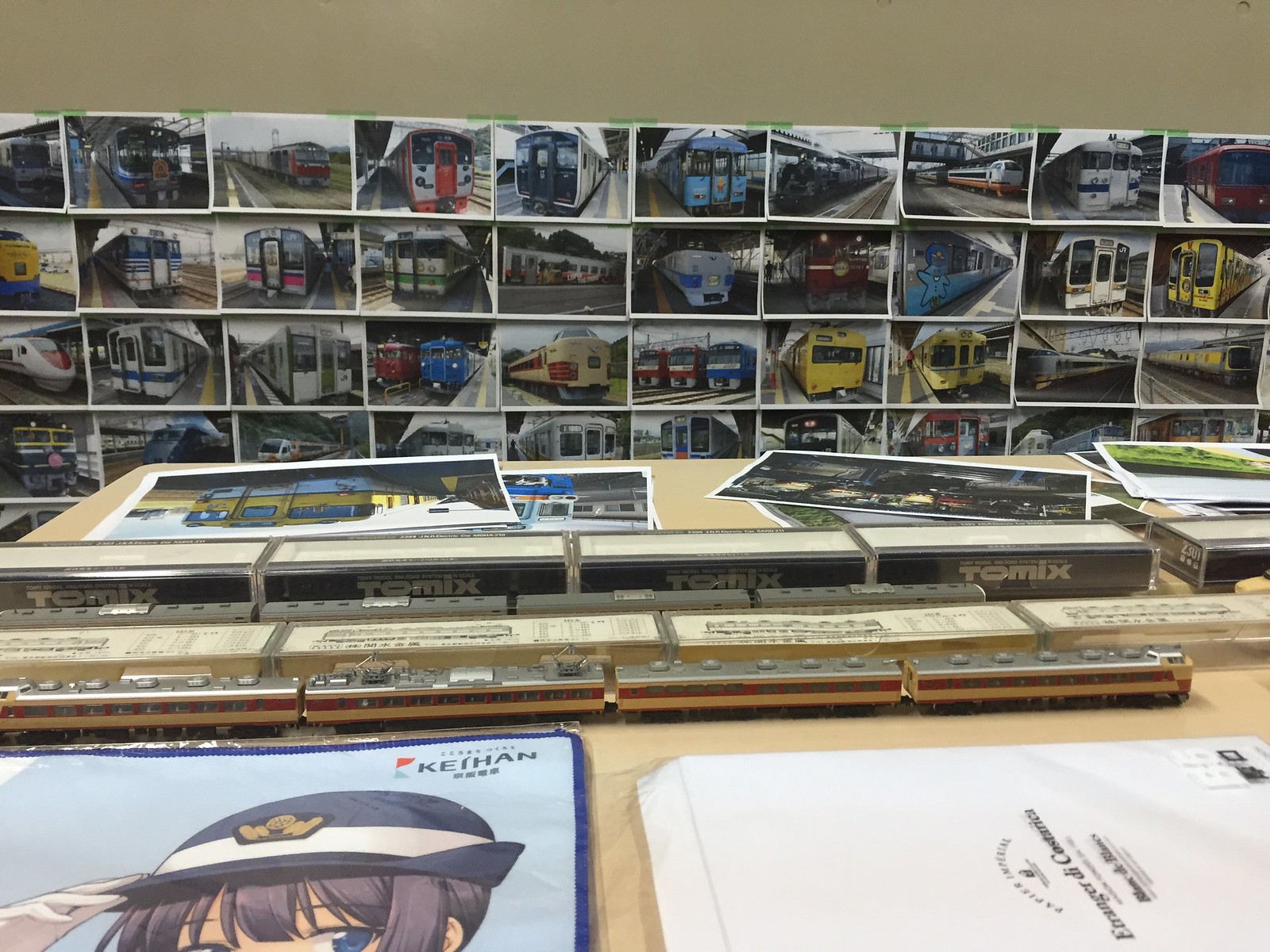This photograph captures an intricate model train display, likely set in a train store, museum, or perhaps an art or photography show. The backdrop features a tan wall adorned with several rows of small, 3x5-inch photographs showcasing various metro train cars, mostly viewed from the rear or side. In the mid-ground, a tabletop displays larger train photos randomly strewn about. Prominently in the foreground, a series of vividly colored yellow and red miniature train cars are linked together, though they are not placed on a track. Additionally, there are boxes labeled "Tomix" which presumably contain more model train components. Among the scattered items on the table, there is also a partial image of an anime character visible, adding a unique element to the scene. The overall impression is that of a dedicated, albeit somewhat cluttered, display by a train enthusiast, where the detailed presentation of model trains and their photographic representations takes center stage.